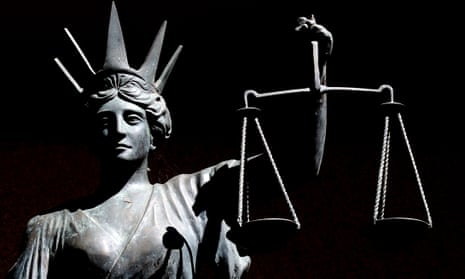The image is a detailed, black and white photograph of a sculpture resembling the Statue of Liberty, but with symbolic modifications. Captured from the bust upwards, the sculpture is set against a stark black background, emphasizing its gray or light porcelain-like features. Lady Liberty is depicted without the traditional blindfold of Justice, signifying a deviation from the notion of impartiality. Instead of raising a torch, she holds a set of balance scales aloft in her left hand, merging the iconography of Justice with that of Liberty. Her distinct starburst crown crowns her head, completing the visual fusion of these two powerful symbols. The interplay of light and shadow in the photograph accentuates the monochromatic contrasts, lending depth and intensity to the striking sculpture.